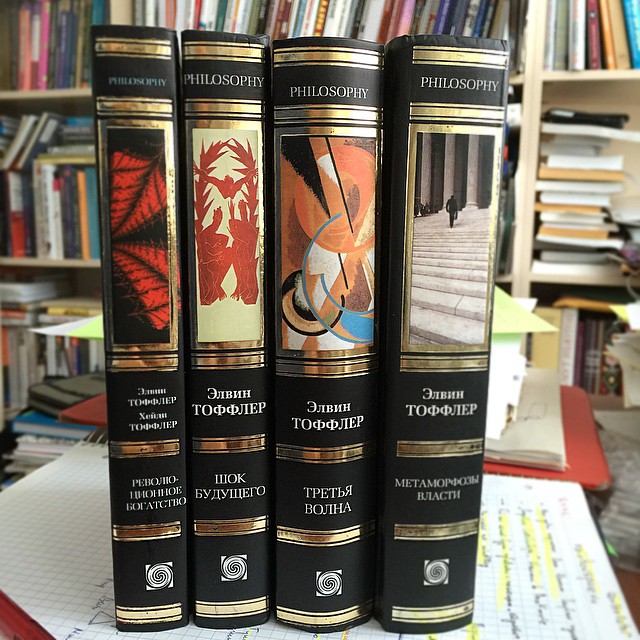The image predominantly features four black books arranged side by side, each adorned with golden accents along their spines. At the very top, all four books display the word "philosophy" in gold. Below this, each book showcases a rectangular golden frame enclosing unique artwork: one book has a striking red and black pattern reminiscent of butterfly wings, the next features a depiction akin to Greek or Roman folk paintings in red and white with three figures, the third is embellished with abstract lines, circles, and colors, and the final book displays a black-and-white photograph of a person ascending steps toward a grand, official building. Beneath these framed images, Cyrillic text indicates the titles and authors' names, also in gold. These books rest on a piece of graph paper with some handwritten notes. The backdrop consists of a slightly cluttered bookshelf, where some books are neatly stacked while others are in disarray, providing a colorful and rich context.